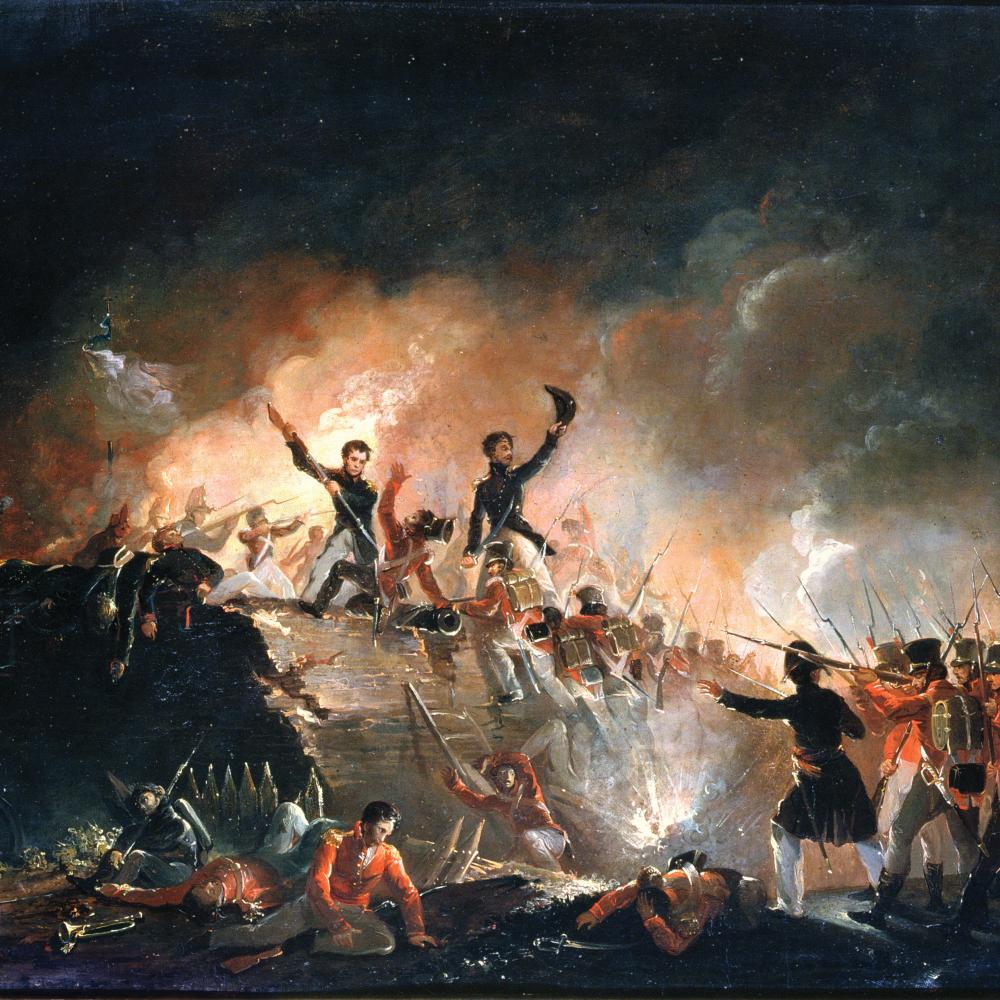This dramatic painting depicts a chaotic night battle scene, likely set during the late 1700s or early 1800s, possibly the Revolutionary War or Napoleonic era. The background is dominated by a dark sky with hints of orange at the bottom, suggesting an explosive battle. The upper portion shows faint white spots resembling stars, while clouds and smoke indicate the ongoing turmoil. In the foreground, a man in a dark-colored coat stands with his back to the viewer, possibly leading a group of soldiers in red coats, identifiable as British troops. These soldiers, armed with rifles affixed with bayonets, advance across what appears to be a river. Nearby, a figure in a blue coat and white trousers, possibly a French or American soldier, is engaged in close combat, stabbing a red-coated enemy with his bayonet. Another soldier raises his tricorn hat amidst the smoky, chaotic battlefield. Explosions and gunfire are evident throughout, with fallen soldiers scattered across the scene, capturing the brutal and chaotic essence of war.